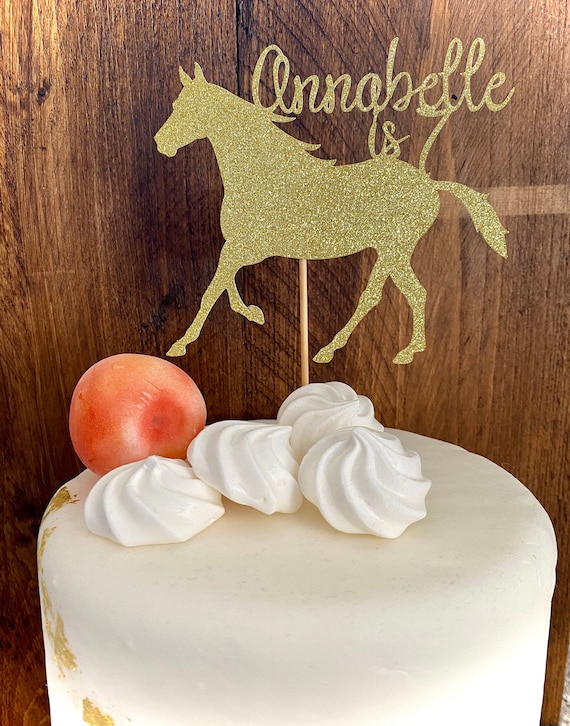This photograph captures a beautifully decorated round cake set against a wooden plank background. The cake is frosted with off-white buttercream icing and features elegant gold leaf decorations on the left side, extending from the bottom towards the top. Atop the cake are four intricately molded white chocolate cookies resembling seashells, artfully arranged in a pile. Nestled among the cookies is a small, uncut, peach-like decoration. A striking golden stick decoration protrudes from the cake, adorned with a gold-flaked horse silhouette. Above the horse, in a cursive script reminiscent of the Disney logo, the words "Annabelle is seven" proudly announce the occasion, marking this as a birthday cake for Annabelle.